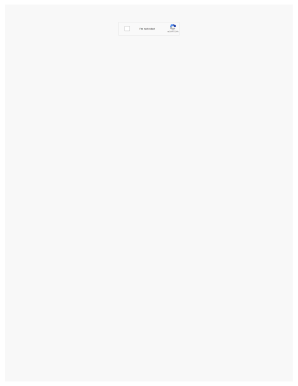The image is a screenshot from a website with a light gray or off-white background. In the upper center area, there is a light gray rectangle outlined with a thin gray line. Inside this rectangle, on the left side, is a small white square with a matching thin gray outline.

To the right of the white square, there is a section of blurred text. Despite the blurring, the word "I'm" is discernible at the beginning, but the rest of the text is unreadable.

Further to the right of the text, there is an almost complete circle, starting with a gray segment at the bottom which transitions into brighter blue and then darker blue shades. Below this circle, there is some text indicating it is a reCAPTCHA logo, although no check marks or additional elements are present within it.

The rest of the page appears blank, void of any additional content or interactive elements.